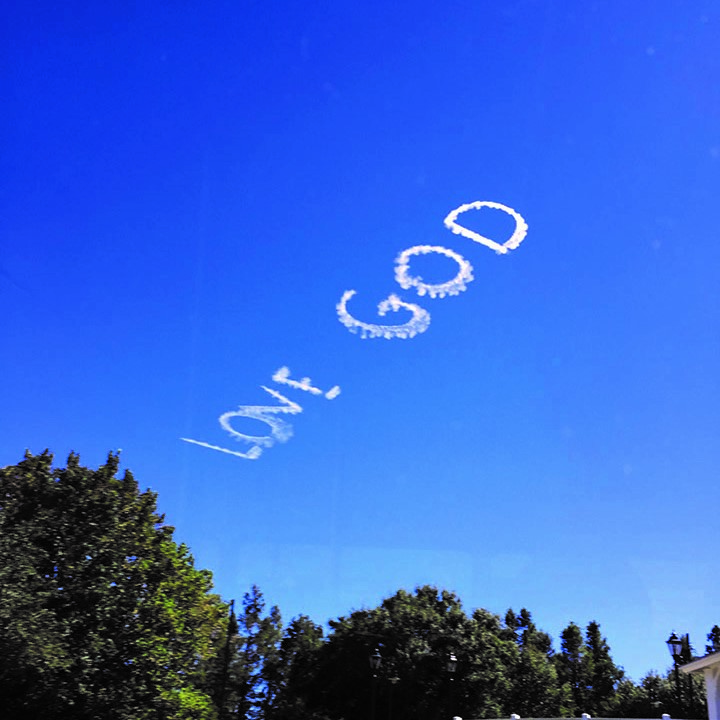The outdoors image captures a vivid, bright blue sky, with a gradient shading from a darker blue at the top to a lighter hue near the bottom. Diagonally across the sky, white smoke letters spell out "LOVE GOD" in all caps, suggesting skywriting done by a plane that is no longer visible. Below this celestial message, the scene transitions to the tops of deep green trees, their leaves dense but not entirely obstructing the sky. On the left, a large tree with dark green foliage dominates, while thinner, taller trees stand to its right. The lower right corner reveals a black streetlight with a glass lantern perched on top, beside a small portion of what appears to be a building with a white roof and siding. The entire scene is bathed in natural light, providing a clear and detailed view of both the skywriting and the lush greenery below.